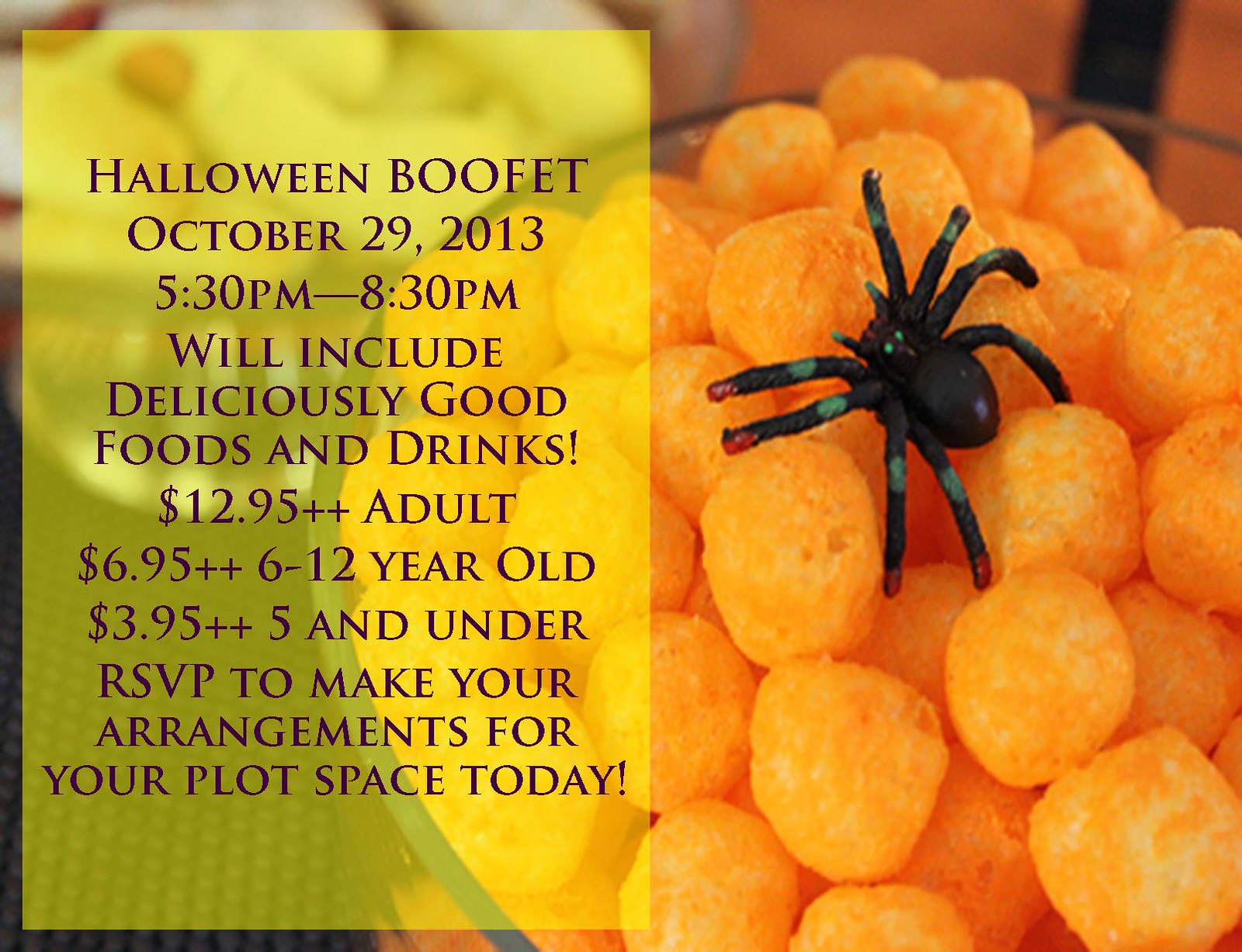The promotional flyer is for a "Halloween BOOFET," a play on words fitting the spooky theme of the event. The event is scheduled for October 29, 2013, from 5:30 p.m. to 8:30 p.m. Attendees can expect "deliciously good food and drinks." The left half of the flyer features a transparent yellow triangle with black text detailing the event information, including the playful Halloween theme and the word "boo" integrated into "BOOFET." Prices are clearly listed: $12.99 for adults, $6.95 for children aged 6 to 12, and $3.95 for kids aged 5 and under. Guests are also instructed to RSVP to secure their plot space, adding a spooky twist to the reservation process. The background of the flyer is a visually engaging close-up image of a table covered with snacks, with the most prominent snack being orange cheese puffs in a clear glass bowl. Atop the cheese puffs sits a black plastic toy spider with red-tipped legs and a green band on each of its eight legs, enhancing the Halloween ambiance.